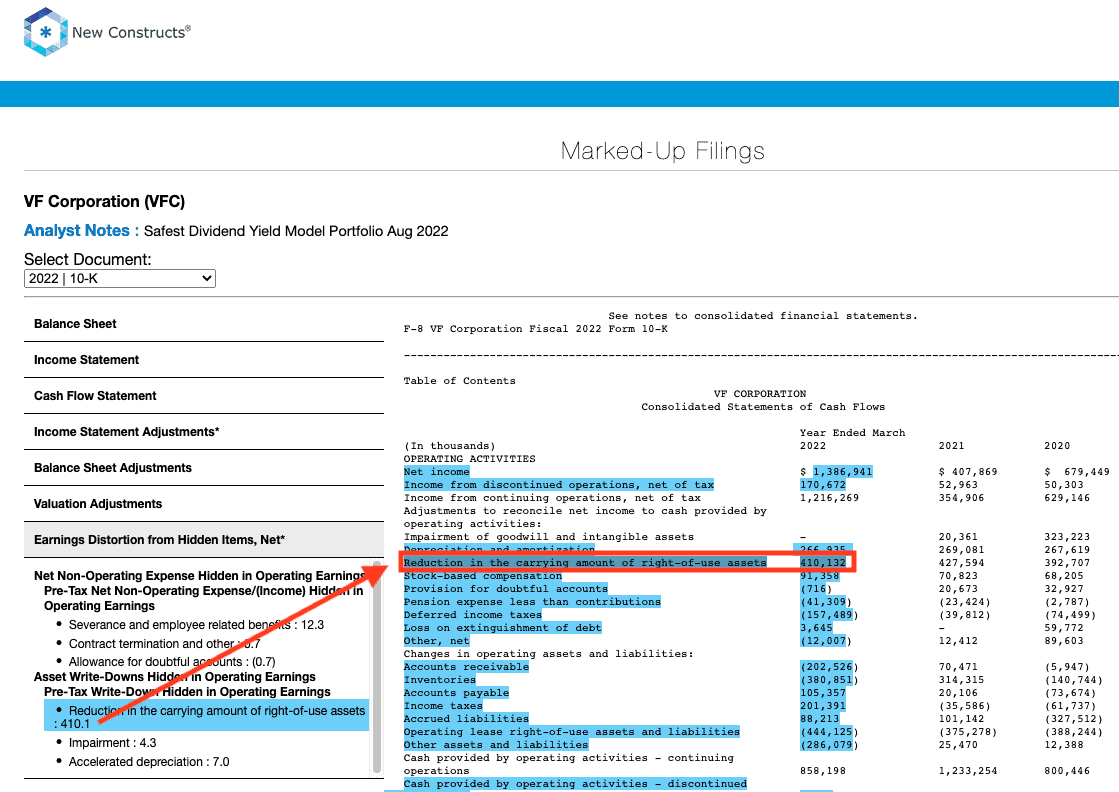In this image, the content is prominently displayed with a screenshot situated in the upper left-hand corner containing the title "New Constructs." Central to the image is a page labeled "Marked Up Fillings." Beneath this section, on the left side, the title "VF Corporation (VFC) Analyst Notes - Safest Dividend Yield Model Portfolio August 2022" is visible. Below this, a dropdown menu labeled "Select Document" shows the option "2022 10-K."

Running down the left-hand side of the page, there is a menu listing several options including "Balance Sheet, Income Statement, Cash Flow Statement, Income Statement Adjustments, Adjustments, Balance Sheet Adjustments, Valuation Adjustments, Earnings Distortion from Hidden Items (Net)." The current selection, "Earnings Distortion from Hidden Items (Net)," is open. Within this section, detailed text describes financial terms such as "Net Non-Operating Expense (Hidden in Operating Earnings)" and "Pre-taxed Net Non-Operating Expense (Income Hidden in Operating Earnings)."

Highlighted in blue with a red arrow pointing towards the right-center of the image is the text "Reduction in the Carrying Amount of Right of Use Assets," which directs attention towards a detailed list of operating activities. This highlight emphasizes the specific financial adjustment being illustrated within the document.